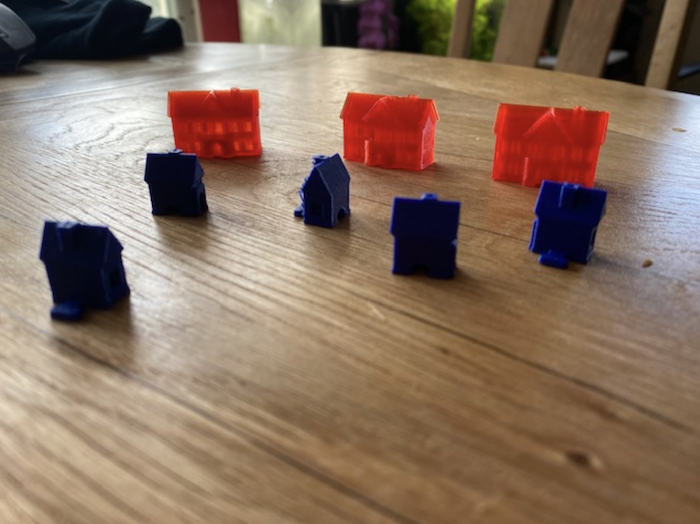The horizontal image captures a scene on a plain wooden table, potentially oak, with 3 red and 5 blue plastic house pieces, reminiscent of Monopoly or Lego houses, arranged towards the center. The red houses, lined up with a notable gleam that gives them the appearance of being illuminated or having lights, contrast against the denser, windowless blue houses set in a slight wavy line. The houses are spread out across the table, which has an assortment of objects including chairs, hinting at a playful or game-related setup, possibly in a dining or game room. Background details like a sports chair are visible, adding context to the environment.